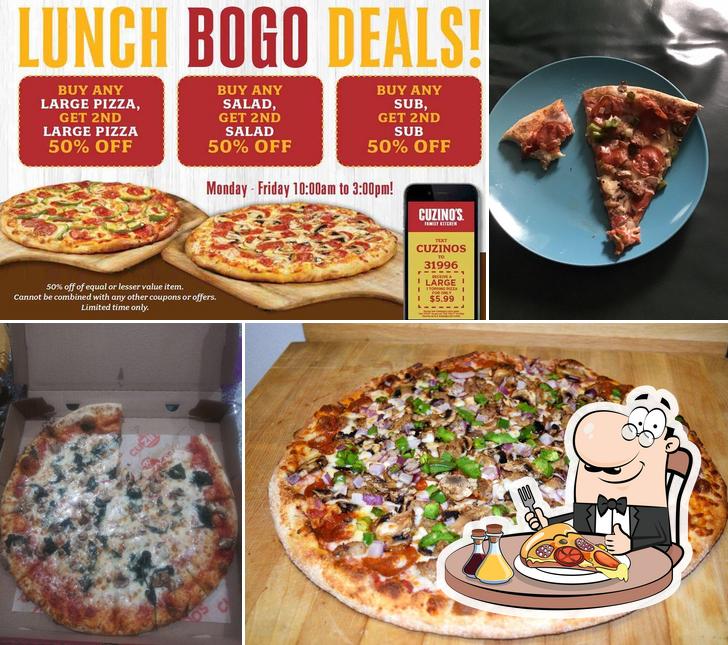Screenshot of the Cuisinos Pizza restaurant webpage, highlighting various features and deals. At the top of the page, there is a prominent banner advertising "Lunch BOGO Deals," available from Monday to Friday, between 10 a.m. and 3 p.m. Below this banner, a series of images showcase the restaurant's offerings:

1. A pair of large pizzas presented on a rustic wooden serving board.
2. A partially eaten slice of pizza on a vibrant blue plate, emphasizing the appetizing nature of the food.
3. A pizza box with one slice missing, suggesting the enjoyment and convenience of takeaway options.
4. A large combination pizza on a wooden table, adorned with a whimsical cartoon figure, presumably representing the Cuisinos logo.

The overall layout and images underscore Cuisinos' focus on delicious, freshly-made pizzas and enticing lunch deals.